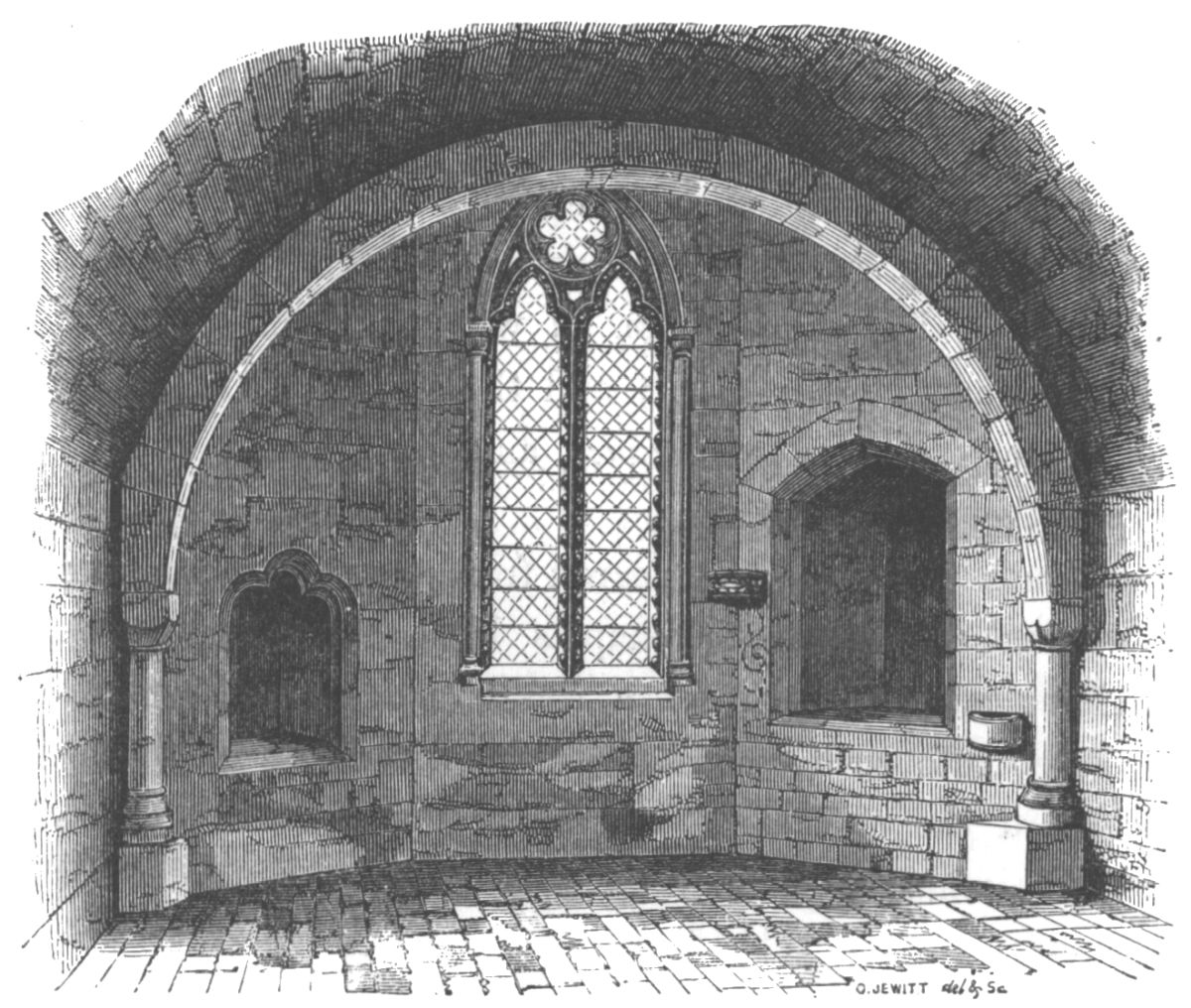This black-and-white illustration, likely a pencil sketch or etching, depicts an interior space that appears to be from an old church or perhaps a fortified structure. The scene features a central, elaborate stained-glass window with intricate patterns and floral grills, bordered by pillars and square platforms. The architectural design showcases a curved, arched ceiling supported by visible stone pillars, with crosshatched shading adding depth to the detailed stone and brick textures of the floor and walls. Flanking the main window are smaller, recessed nooks that resemble decorative fireplaces or storage alcoves, though their exact purpose is ambiguous. The entire composition exudes a sense of historical elegance and detailed craftsmanship.